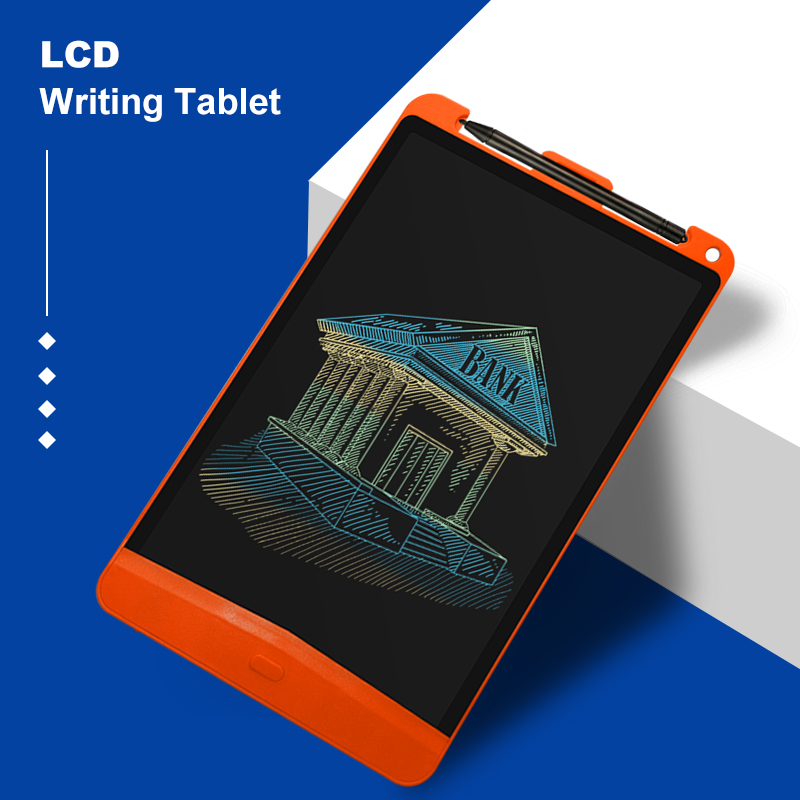In this promotional image, a red writing tablet with an orange bezel and black screen is prominently displayed, leaning to the right against a white block. The tablet features a black pen clipped at the top, resembling a stylus. The screen displays a multicolored sketch of a classical bank with a triangular roof, columns, a grand staircase, and a large door, rendered in blue, green, yellow, and orange. The tablet has a button at the bottom center and a hole in the top right corner. In the upper left corner of the image, on a blue backdrop, bold white text reads "LCD Writing Tablet." Below the "W" in "writing," a vertical white line extends downward, followed by four vertically aligned white diamonds. The overall background alternates between blue and white, enhancing the focus on the tablet and its features.